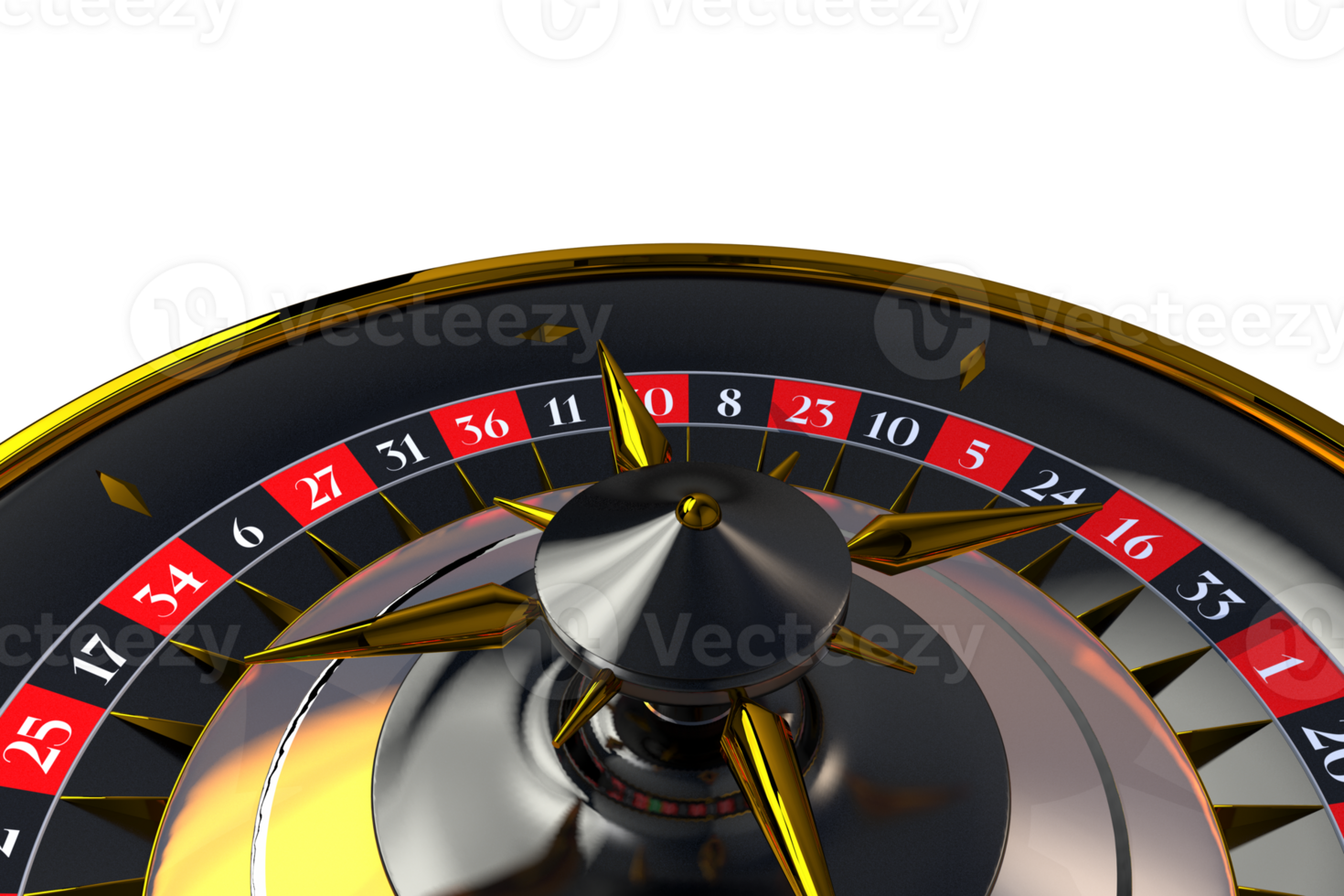The image features a detailed view of a rectangular, horizontal roulette wheel. The outer rim of the wheel is gold, while the inner section is black. The wheel itself is the standard type used in gambling, characterized by alternating red and black numbered spaces. The numbers on the wheel include 25, 17, 34, 6, 27, 31, 36, 11, 10, 8, 23, 10, 5, 24, 16, 33, and 1, all displayed in white font. Each number is set within either a red or a black square, creating a striking visual contrast. The center of the wheel features a black, slightly pointed circle. The dials on the wheel are also gold, adding to the luxurious appearance.